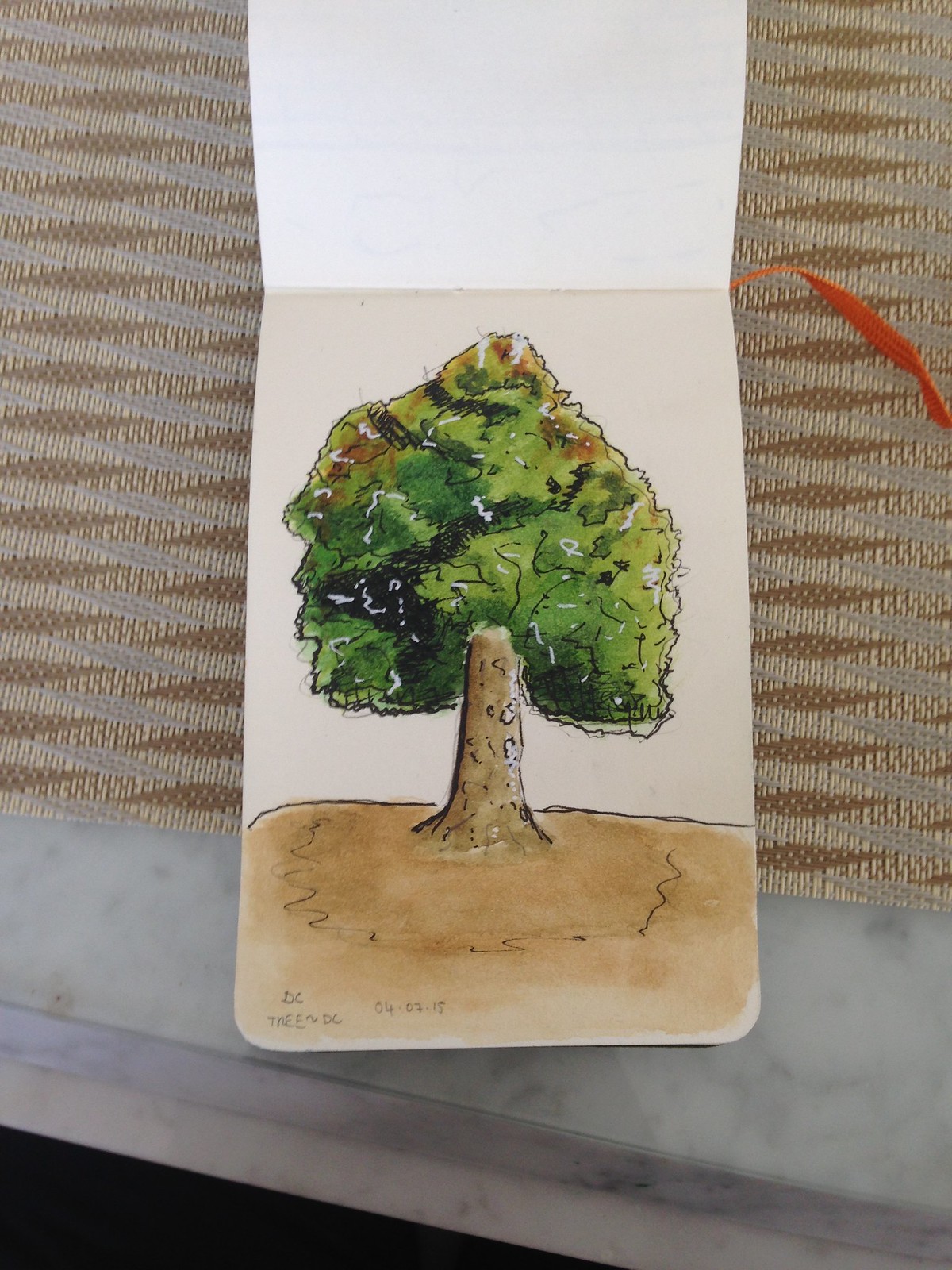An open sketchbook is displayed on a marble table adorned with a tan and brown textile tablecloth. The sketchbook, opened to a portrait-oriented page, features a detailed watercolor and ink drawing of a solitary tree. The tree, rooted in a small patch of brown earth against the white background of the paper, boasts a sturdy brown trunk that extends into a lush green canopy. The opposite page of the sketchbook is folded up, revealing only a faint glimpse of its blank backside.